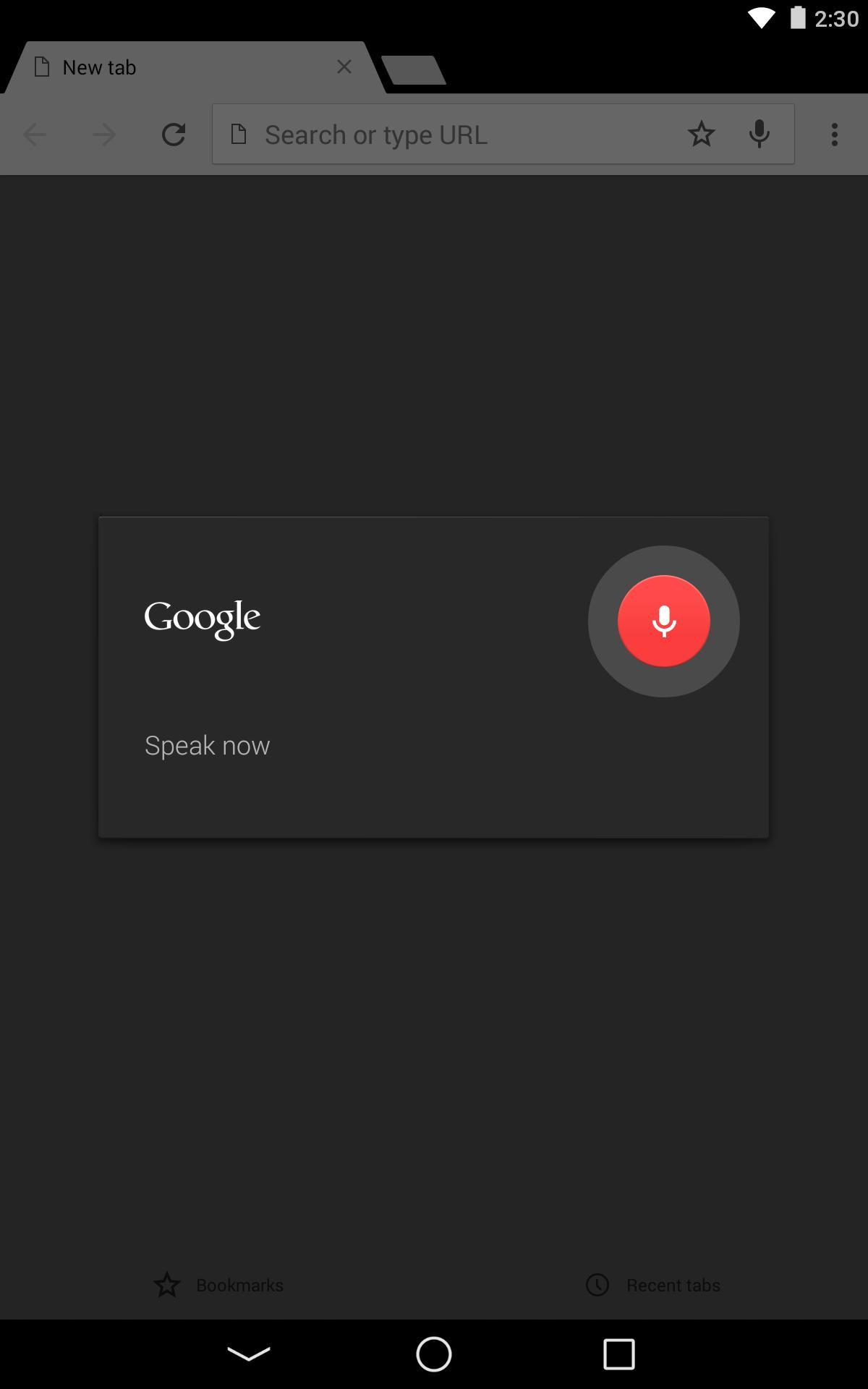The image depicts a screenshot of a smartphone screen in dark mode. At the top right corner, the white icons include the Wi-Fi signal, a battery status indicator, and the time displayed as 2:30. Below, a gray-bordered "New Tab" bar appears with a small piece of paper icon on the left and an 'X' on the right to close the tab. Directly under this, there is a backward navigation arrow, followed by a search bar that reads "Search or type URL." The search bar features a star, a microphone icon, and three vertical dots on the right side.

Taking up a significant portion of the screen is a large black area. Superimposed on this is another black rectangle showcasing the Google logo in its standard white font. Beneath the logo, there is a round black button with a red circle in the middle and a white microphone icon, accompanied by text in a lighter white that reads "Speak now," indicating voice input functionality.

The bottom part of the screen features three icons: a downward-pointing arrow, a round home button, and a square, which are standard navigation buttons on many smartphones. The overall screen presents the interface of a mobile browser in dark mode, ready for a voice search input.